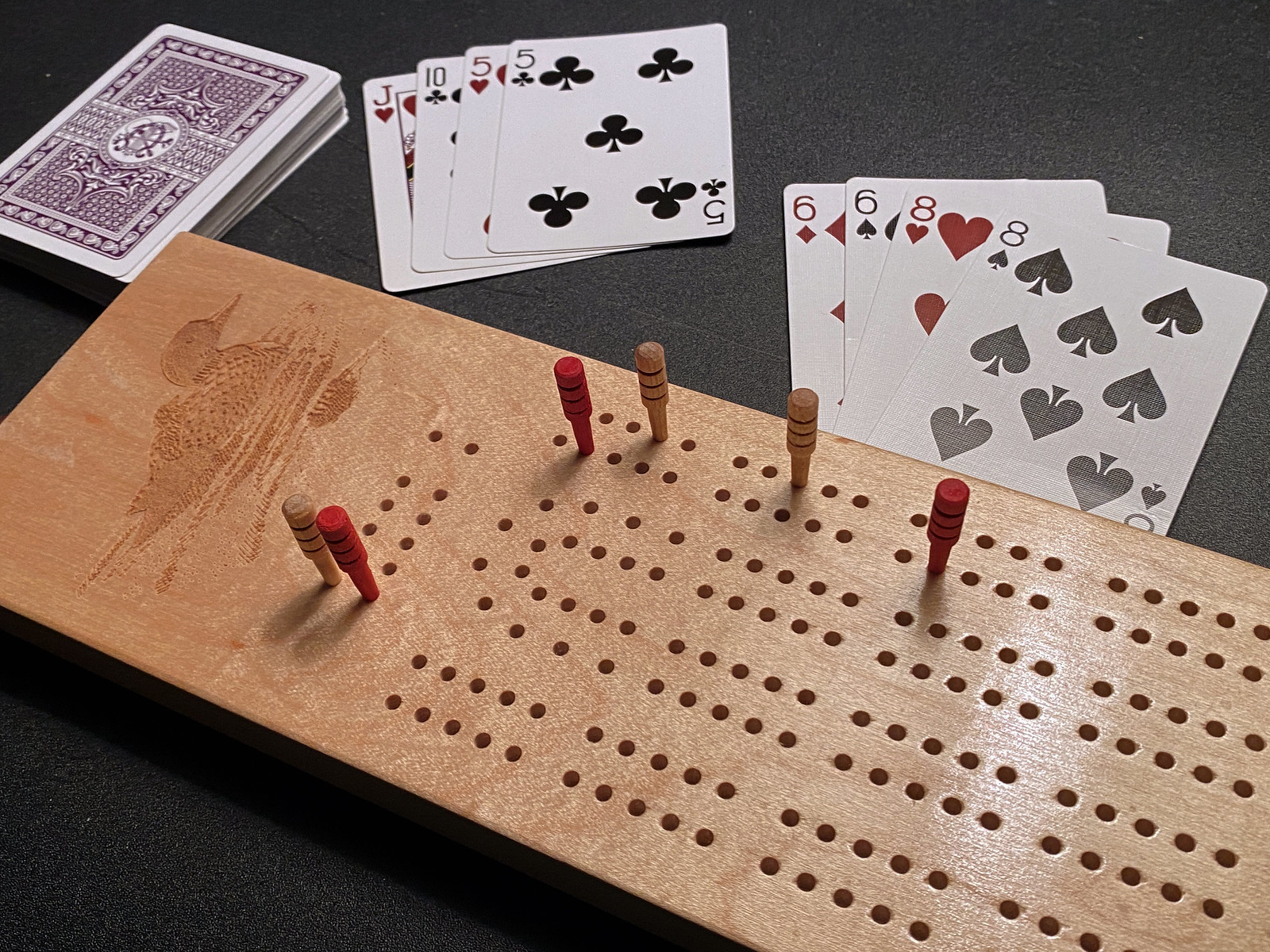This image depicts a rectangular wooden board game, intricately crafted with a carving of a duck at the top. The game board features a grid of holes, organized into two horizontal rows at the top and multiple vertical rows below, each consisting of three layers of holes. These holes are designed for wooden pegs, currently occupied by three red pegs and three brown pegs positioned at various points on the board. To the right of the game board, a set of playing cards is laid out, showing four upright cards at the top: a jack, a ten, and two fives. Nearby, another cluster of four cards displays two sixes and two eights. Additionally, a stack of face-down playing cards rests beside them, completing the scene of this intriguing wooden board game setup.